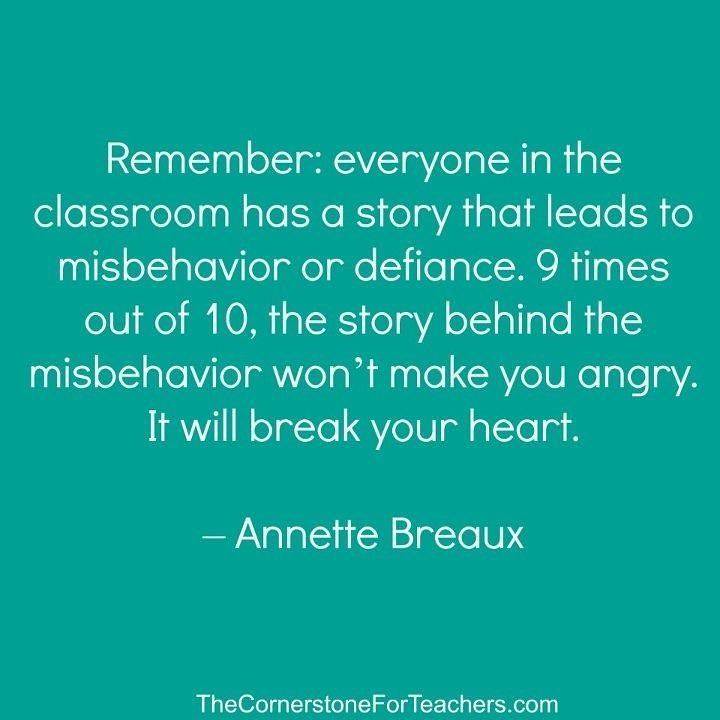The graphic depicts an inspirational message set against a light seafoam green background, with white text emphasizing empathy for students' behaviors. The central quote reads, "Remember, everyone in the classroom has a story that leads to misbehavior or defiance. Nine times out of ten, the story behind the misbehavior won't make you angry. It will break your heart." This quote is attributed to Annette Breaux and is sourced from TheCornerstoneForTeachers.com. The slide likely serves as a resource for educators, aimed at fostering understanding and compassion in classroom management. The background's simplicity, featuring only text without additional imagery, underscores the importance of the message.